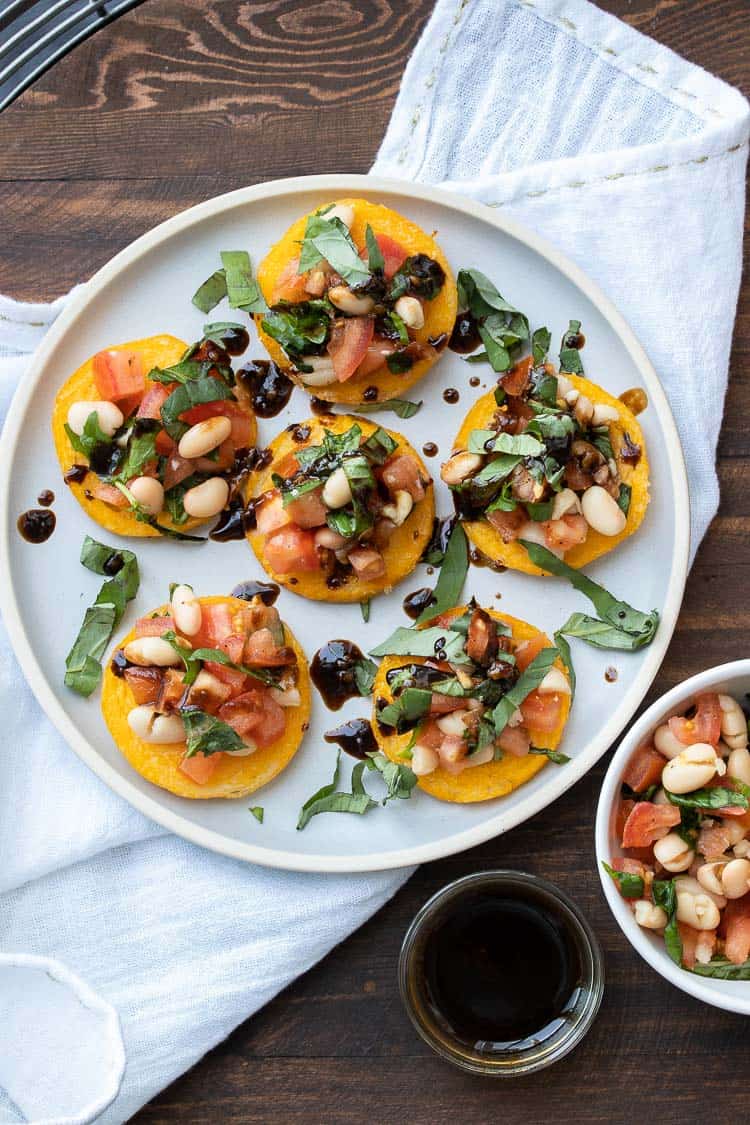The image depicts an overhead shot of a dish from a restaurant, featuring six round, orange slices of a vegetable—possibly tomatoes—beautifully arranged on a white plate placed atop a white linen napkin. Each slice is garnished with a medley of beans, chopped tomatoes, and a leafy green, likely basil or celery, with a drizzle of either soy sauce or balsamic vinegar enhancing the presentation. Accompanying the dish is a small cup of sauce for dipping, likely containing soy sauce or balsamic vinegar, and another cup filled with additional toppings of beans and tomatoes. The table beneath the setting is made of dark wood, providing a rich contrast to the crisp, white dishware.